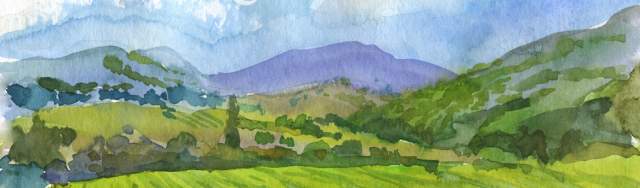This watercolor painting captures a serene landscape with an illustrative style. The scene is primarily cool-toned, dominated by greens, blues, and pale purples, with an overarching rustic farmland feel. In the foreground, there are lush green fields, dotted with darker greens representing bushes and clusters of forested areas. Among the greenery, low-lying shrubs and pine trees can be seen, adding depth and texture. The middle ground features golden hills, their slopes adorned with additional foliage and small trees. Ascending from the center to the top right corner is a prominent mountain. In the background, distant mountains appear in shades of blue and violet, creating a layered effect. The sky above is a pale blue, streaked with wisps of white clouds. The entire composition is set within a long, thin horizontal rectangle, designed to capture broad strokes and the essence of the natural elements rather than fine details. The painting exudes a dreamy daytime atmosphere, devoid of animals or human presence, focusing solely on the beauty of nature.